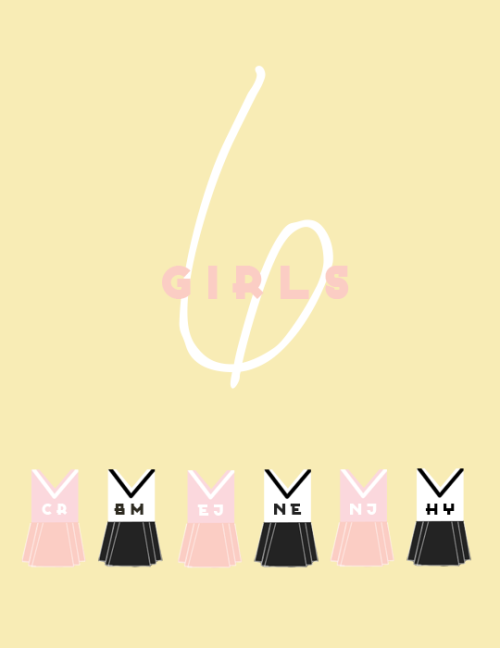The image appears to be an advertisement or poster featuring six cheerleader outfits depicted graphically. The background is a beige or pale yellow color with a stylish white curved shape at the top displaying a large white number "6." Above this number in pink, bold letters, it reads "GIRLS." The cheerleader outfits are arranged in a rotating pattern of pink and black/white designs. Each outfit consists of a ruffled skirt paired with a coordinated, v-neck top, all marked with different letters. From left to right, the uniforms are: pink with "CR", black and white with "BM", pink with "EJ", black and white with "NE", another pink with "NJ", and finally, black and white with "HY." This visually appealing display might be promoting a K-pop girl band or similar group.